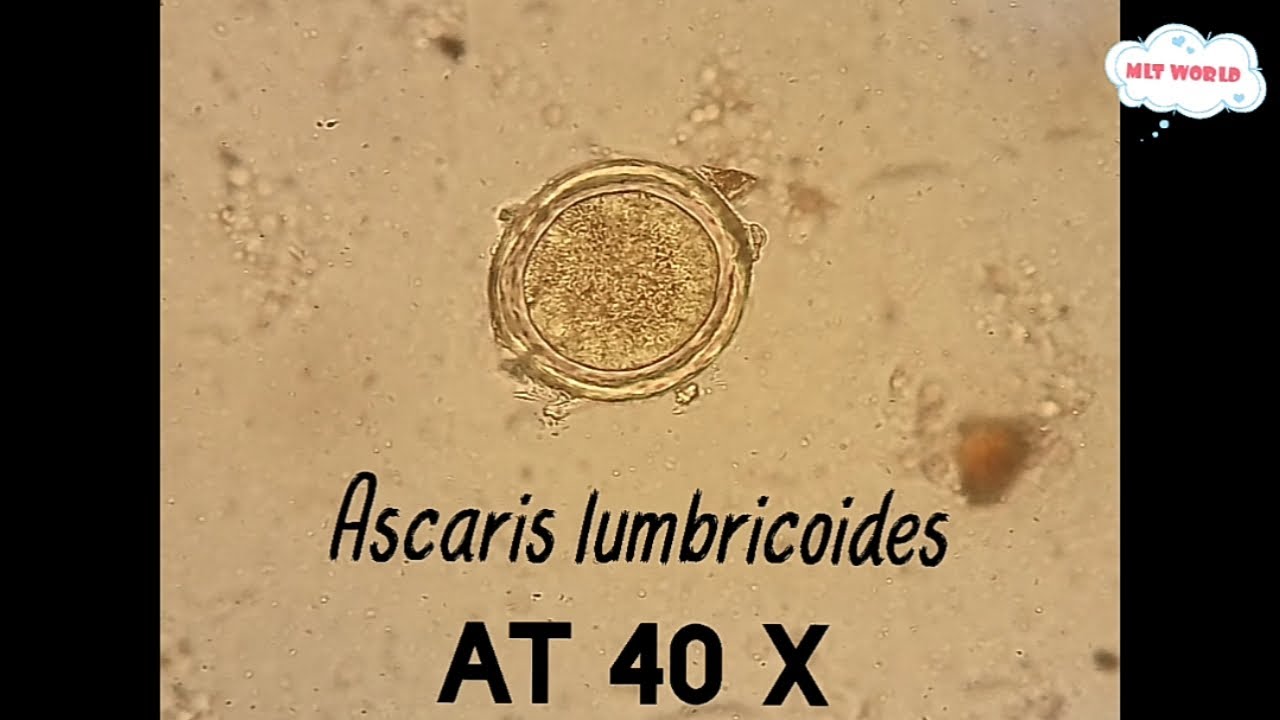This color slide photograph, oriented in landscape, is bordered on the left and right by narrow vertical black strips. The central image features a detailed microscopic view against a dark beige background. Prominently displayed in the center is an elliptical cell, identified as Ascaris Lumbricoides. The cell's structure includes a visible cell wall encasing a rough, grainy interior surface. Additional indiscernible objects float in the background. Beneath the cell, in black handwritten text, is the label "Ascaris Lumbricoides," followed by "AT40X," indicating the magnification level of forty times. In the upper right corner, a white cloud with blue highlights contains the red text "MLT World."